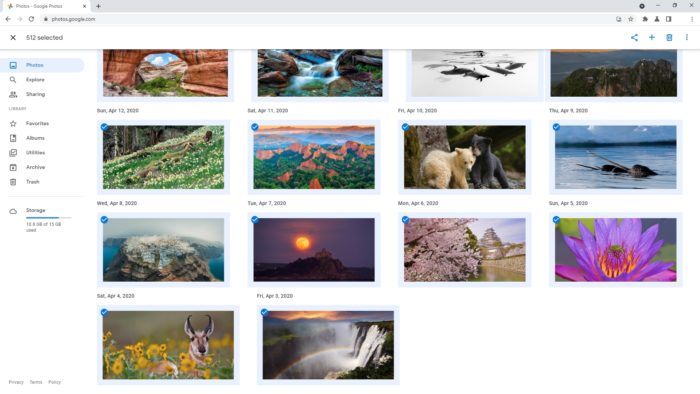This image is a screenshot of an open website page in an internet browser, specifically Safari. The browser window features a single open tab displaying the URL, photos.google.com. At the top of the window, there's a gray bar with the recognizable Apple icon to the extreme left.

Below the browser bar, the Google Photos interface is visible. At the top of this section, the interface indicates "512 selected," positioned next to a black 'X' icon on the left. To the right of this selection count, there are icons for sharing, adding items, and managing account settings; these icons include a share icon, a plus sign, and a blue square with a white mannequin head in the center.

On the left sidebar of the interface, menu options are listed in vertical order, which are: Photos, Explore, Sharing, Favorites, Albums, Utilities, Archive, and Trash.

The central part of the screen showcases a grid of thumbnail images, representing a variety of landscape and nature-themed photos. These images include:
1. A plateau.
2. A waterfall.
3. A shark swimming.
4. A mountaintop.
5. Deer in a field.
6. An aerial view of mountains.
7. Two bear cubs playing together.
8. Narwhals breaching from the ocean.
9. A picturesque sunset.

Each image appears to be a high-quality, generic wallpaper suitable for various digital backgrounds.